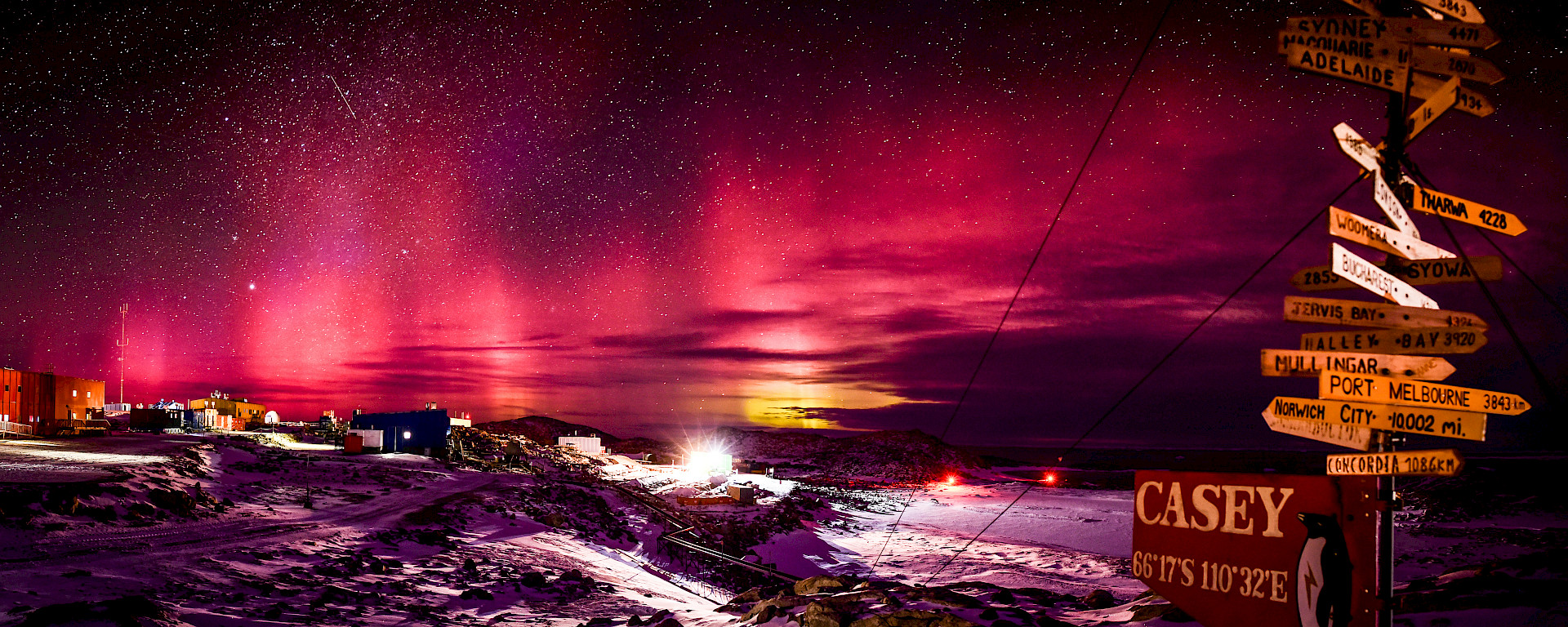A vibrant panoramic aerial view reveals a mesmerizing landscape bathed in shades of pink and purple, with dark black to purplish hues at the top speckled by numerous white dots, likely stars. Prominently, a bright pink band stretches across the center, accentuated by bursts of light piercing through. On the right side, a wooden post brims with an assortment of street signs, each pointing to various cities: Concordia, Norwich City, Port Melbourne, Mullinger, and more, all mounted on a single pole, totaling about a dozen signs. Amongst them, a larger sign marked "KC" features the coordinates "66 degrees 17' south, 110 degrees 32' east," adorned with a small painting of a penguin. Below, snow blankets the ground around this illuminated post, with lights from the ground casting a soft glow on the snowy landscape. Slight hills are scattered with buildings arranged in a row, enhancing the picturesque scene. In the background, a port area is illuminated, with boats dotting the water, and distant structures marking the horizon. The overall clarity of the image is striking, with natural light enhancing the vivid colors and detailed features.